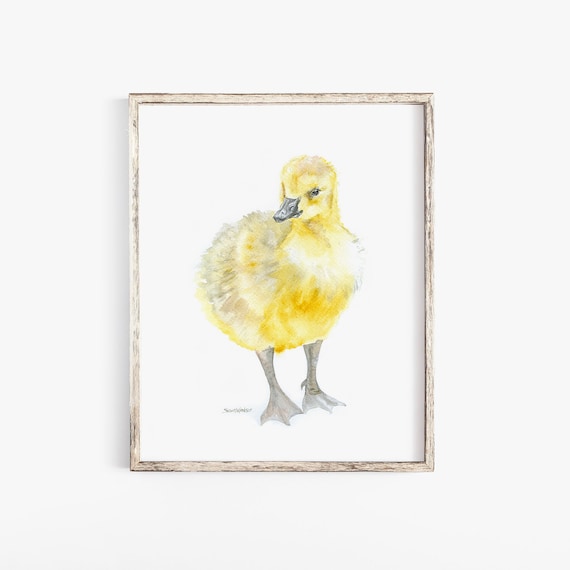The image depicts a framed painting of a small, realistic duckling positioned against a white background. The frame is constructed of wood. The duckling, primarily a bright yellow with multiple shades including light and dark yellow, as well as touches of gray and black, appears very fluffy and detailed. Its down feathers and body showcase variations in color, enhancing the realistic feel. The duckling’s stubby beak, webbed feet, and beady eyes are all a dark grey, adding depth. The painting highlights the duckling’s delicate and peaceful appearance with subtle streaks of white for added detail, presenting a charming, lifelike depiction of the animal.